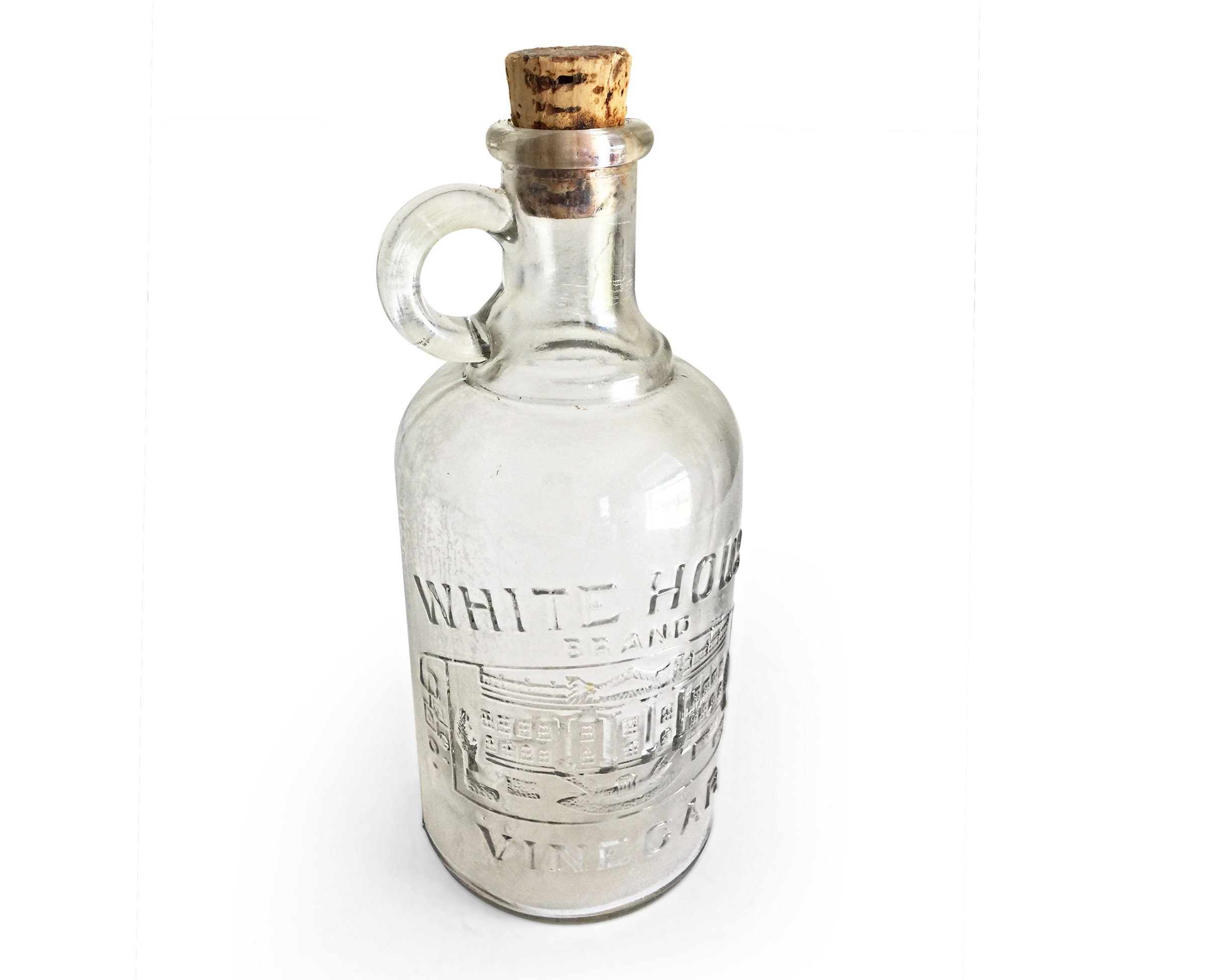This image features a vintage, clear glass bottle reminiscent of old-style Canadian maple syrup or liquor bottles. The bottle has a wide base making up about 70% of its height, which then sharply tapers into a narrow neck. On the left side of the neck, there's a small circular handle that looks worn, ideal for looping a finger through. The cork stopper at the top appears quite aged. The bottle is adorned with raised, embossed lettering and imagery: it prominently displays 'White House Brand' across the front with an etched illustration of the White House below it, followed by the word 'Vinegar'. The photo is presented against a white background, emphasizing it as a product image. The glass also reveals a seam line beneath the handle, a testament to its older manufacturing process. Faint reflections hint at a window to the right and shelves to the left, while the bottom of the jug shows some dirt, adding to the vintage feel.